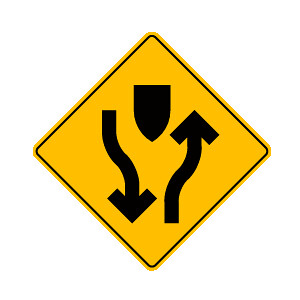The image displays a slightly blurred, yellow diamond-shaped road sign with a black border around its edges, set against a white background. In the center of the sign, there's a black shield-like symbol that features a squared top and tapered bottom. Flanking the shield are two prominent, curved arrows: the left arrow curves from the top left down and then inward toward the center, while the right arrow starts from the bottom right, curving upward. The sign appears to indicate that traffic should split and navigate around a divider, suggesting the presence of an obstruction or a hill in the middle of the road. Surrounding the image are artifacts, implying the sign has been cut out from a larger context.